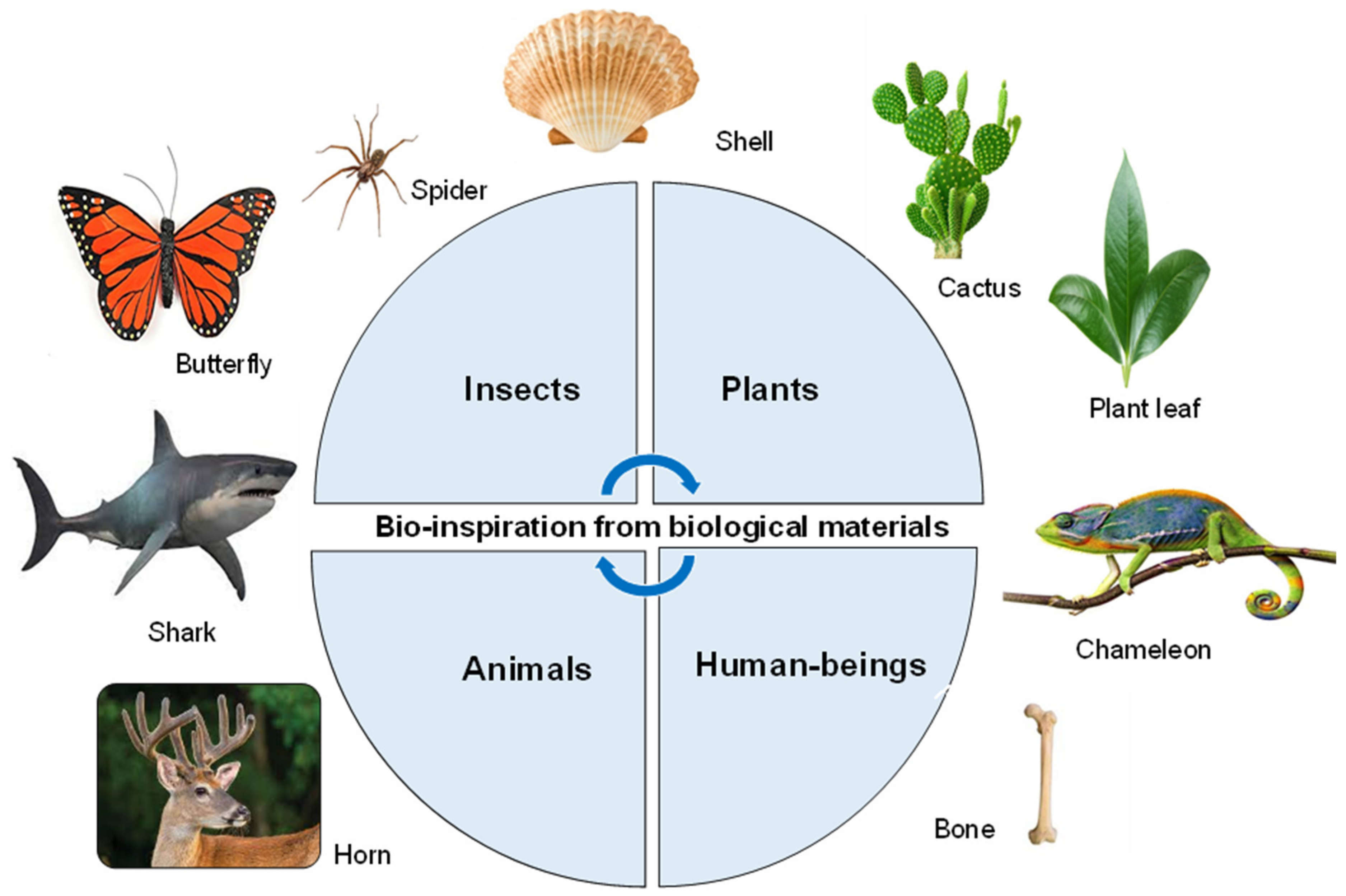The image depicts a detailed diagram titled "Bio-Inspiration from Biological Materials." At the center of the diagram is a circle, evenly divided into four quadrants. Each quadrant is labeled: "Insects" (upper left) in black text, "Plants" (upper right), "Animals" (lower left), and "Human Beings" (lower right). Blue arrows inside the circle connect these categories, with semicircles linking insects to plants, and human beings to animals.

Surrounding the circle are various images linked to their respective categories. At the top are a shell and a cactus, next to which is a plant leaf. Moving right, the diagram shows a chameleon and a reindeer, followed by a bone at the bottom which represents human beings. To the left, there's a shark and other examples including a butterfly and a spider associated with insects.

The chart's background is a light blue color, enhancing its colorful and visually engaging design. Each image icon around the circle complements the biological category it represents, creating an intuitive and informative visual representation of bio-inspiration derived from different biological sources.